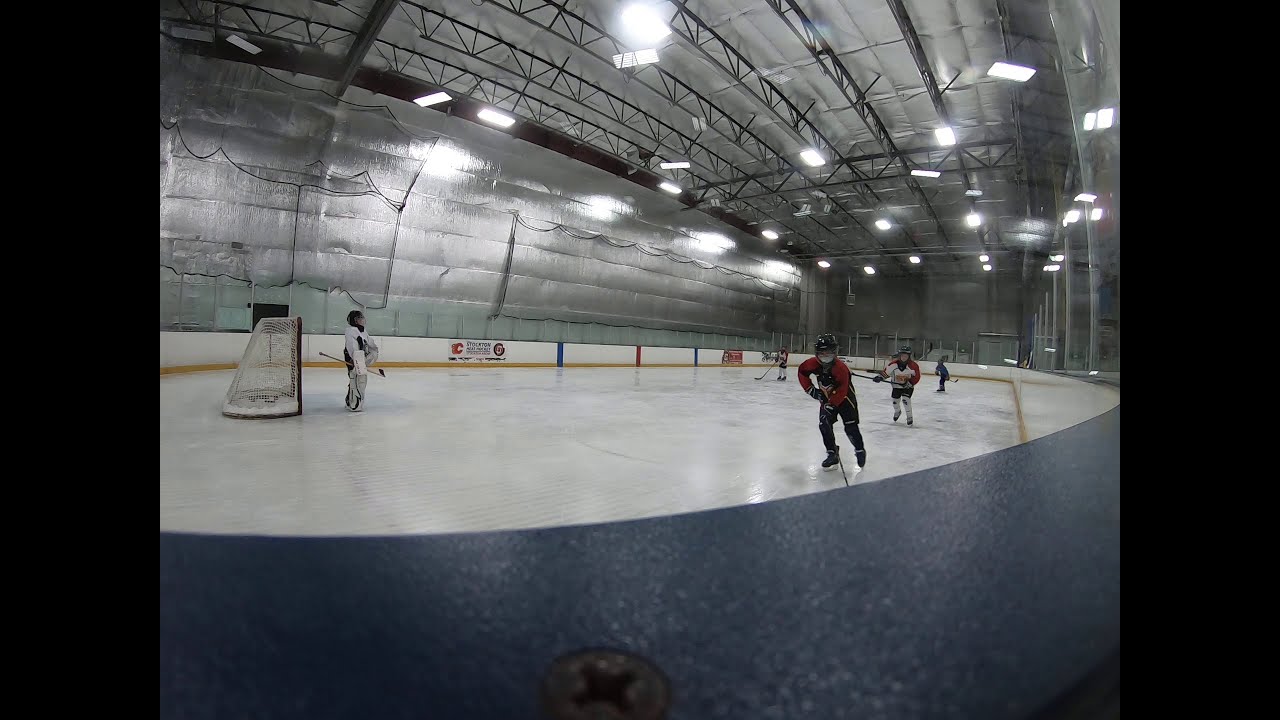The photograph captures an indoor ice hockey rink, taken from a spectator's perspective near the railing. The image shows five skaters on the rink, indicating a game in progress. Two players are in red uniforms, and two are in blue, while one player in the far corner wears a red and white uniform. Central to the composition is a goalie in front of the net, indicating the rink's left side. The player in the foreground, wearing red, has their stick poised, suggesting imminent action. The ice rink has an oval shape, with a protective screen around the perimeter and multiple fluorescent lights illuminating the scene. The far wall of the rink is plain, and two indistinct banners hang on the opposite side. Overall, the image conveys an active moment within a spacious, undecorated ice facility designed to minimize echo.